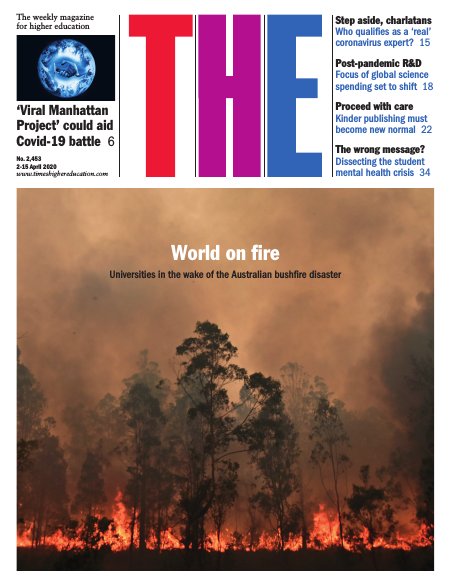**Caption:**

The image is from a news publication titled "The Weekly Magazine for Higher Education." The publication is divided into two main sections, with the text appearing at the top and an image at the bottom.

### Top Section:
On the upper left corner, the text "The Weekly Magazine for Higher Education" is prominently displayed. Below that, there's an image of blue sound waves set against a black background. Beneath this image, a headline reads: "Viral Manhattan Project Could Aid COVID-19 Battle." Additional details include the issue number "2485," date "15 April 2020," and a URL to timeshighereducation.com, along with the number "6" to the right of the headline.

Adjacent to these details, the magazine's acronym "T H E" is stylized with the letters colored in red, purple, and blue respectively. Below this, a list of articles with hyperlinks is provided:
1. "Step Aside Charlatans" - Who qualifies as a real coronavirus expert? (15)
2. "Post Pandemic R&D" - Focus of global science spending set to shift (18)
3. "Proceed with Care" - Kinder publishing must become the new normal (22)
4. "The Wrong Message" - Dissecting the student mental health crisis (34)

### Bottom Section:
The lower section features an impactful image capturing the Australian bushfires. The photo shows a forest engulfed in flames, with dark smoke filling the sky. Superimposed on this dramatic scene, the text reads: "World on Fire." Beneath this, another caption states, "Universities in the Wake of the Australian Bushfire Disaster," illustrating the widespread destruction and the subsequent impact on academic institutions.

This detailed composition provides a vivid and informative snapshot of pressing global issues and their implications for higher education.